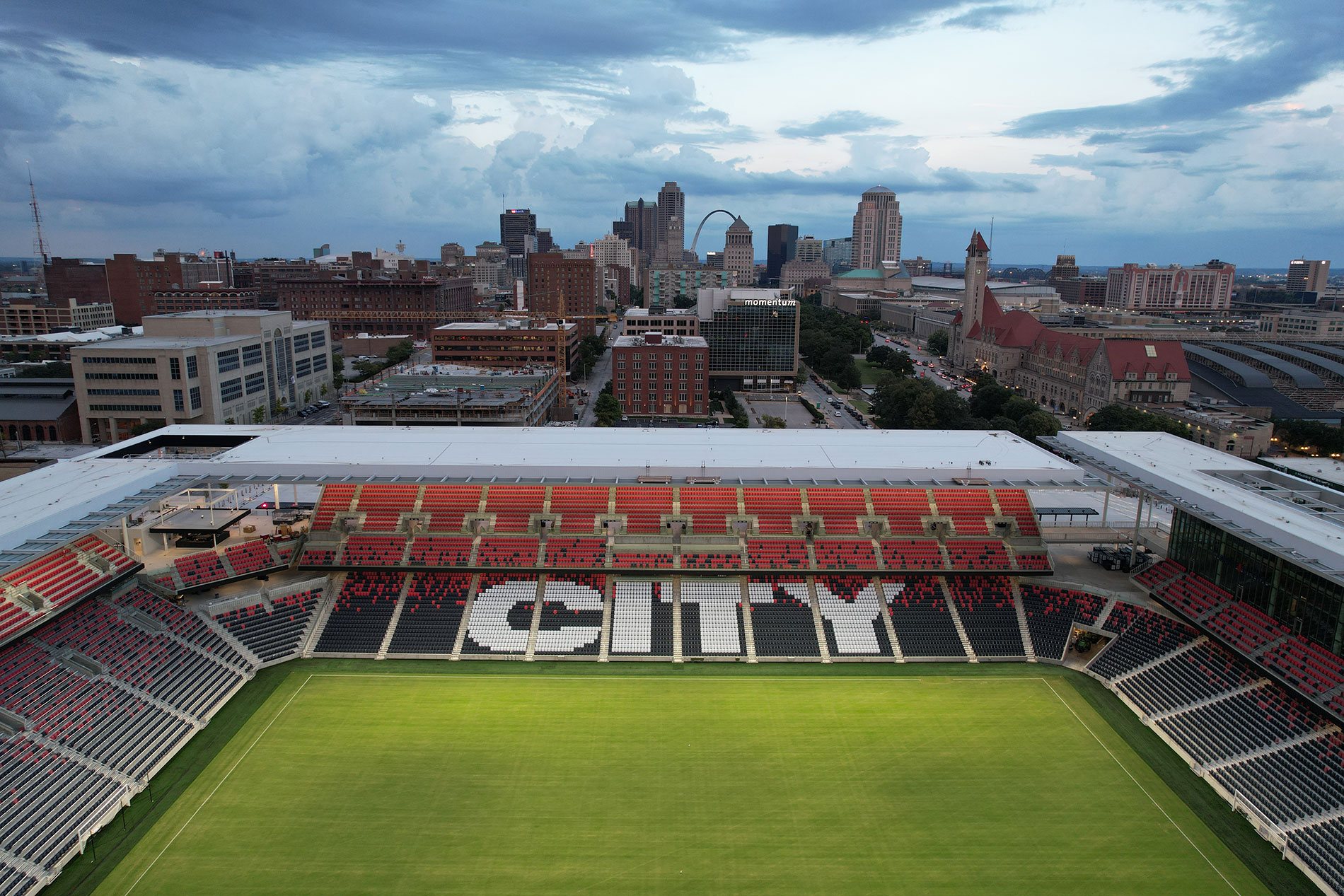This photorealistic image captures a high aerial shot of an empty stadium foregrounded against a metropolitan cityscape. The lower half of the photograph is dominated by the stadium, showcasing a radiant green grass field without any goalposts or distance measuring lines, making the specific sport unclear. The stadium seating, characterized by white aisles interspersed with dark blue and red seats, forms the word "City" prominently in white. The three visible sides of the stadium encompass the bright field, while the closest side is not shown due to the image's elevated and angled perspective. Above the stadium, the upper half of the image features a sprawling urban landscape with an array of mostly short buildings, a few slightly taller structures, all with multiple windows. The sky overhead is predominantly cloudy gray, with a small patch of clear sky visible on the right, casting an overcast light over the city and stadium. The overall ambiance of the scene is a somewhat dark yet vivid representation of both the architectural and urban elements in the frame.